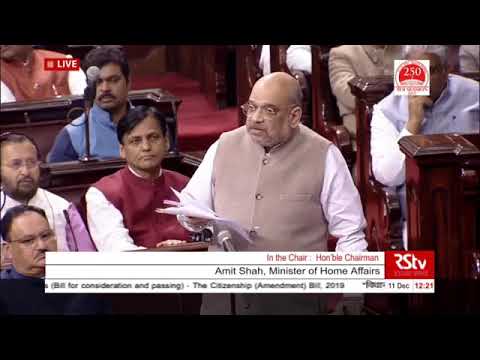The image is a screenshot of a live TV broadcast from a parliamentary setting, featuring rows of wooden pews and various individuals who appear to be Indian. At the center is an older, bald man with medium-dark skin, standing at a lectern with a microphone in front of him. He is wearing a beige high-collar vest with several buttons over a long-sleeve white shirt and holding a stack of papers. The red "LIVE" icon is displayed at the top left, and to the right, the label "RSTV" is visible. Below him, a caption reads: "In the chair, Honorable Chairman, Amit Shah, Minister of Home Affairs." The scene is set against a backdrop of red carpet and people in a variety of colorful attire, including red, purple, blue, and tan.